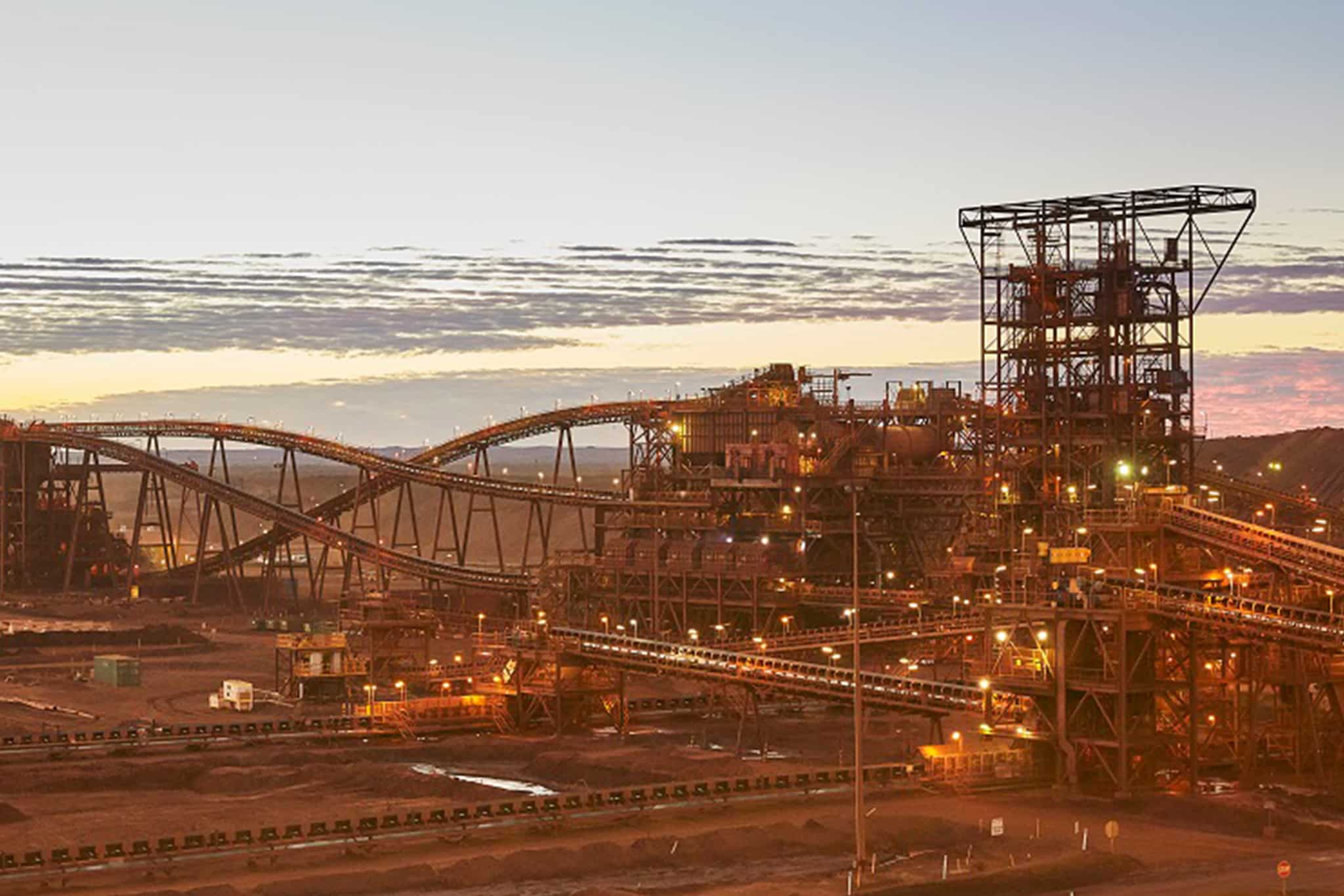The image depicts an industrial rail yard, likely a part of an ore processing or oil refinery plant. The scene is set under a grayish-blue sky filled with wispy clouds, indicating early morning or dusk. The top half of the photo largely showcases these clouds, contributing a hazy atmosphere to the image. Dominated by earthy brown and black tones, the foreground is filled with an intricate network of conveyor lines leading down to the rail yard, where ore carts can be seen. To the right, a prominent tower structure, partially shrouded in scaffolding, is under construction. This tower resembles a flare or exhaust tower, further emphasizing the industrial nature of the scene. Numerous lights scattered throughout the area enhance the industrial look, illuminating bridges and train tracks that lead underneath the industrial superstructure. The entire area is dirt-paved, adding to the rugged, functional aesthetic of the facility.